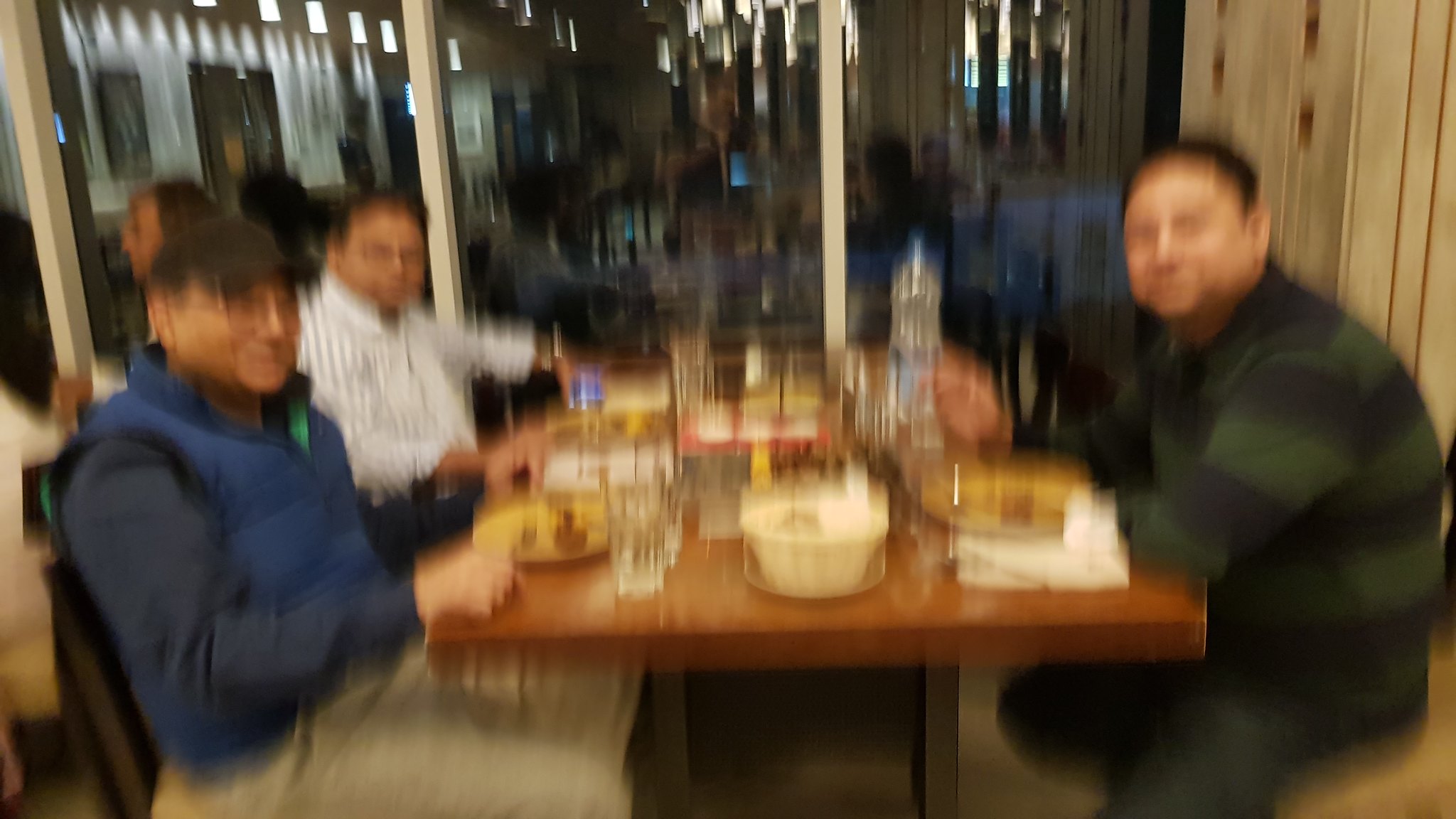This blurry color photograph depicts three men seated around a thick, dark brown wooden table with tan cushions, inside a restaurant adorned with yellow plates and silverware. The men are enjoying a meal laden with an array of food and drinks, including clear glasses and a large bottle, possibly water, placed on the edge of the table. The first man on the left, wearing a blue shirt with a matching blue vest, tan or gray pants, and a black hat, is captured in conversation. He also wears glasses and has a brown-toned complexion. Next to him, the second man, dressed in a white and black striped shirt with dark pants and glasses, has brown skin and black hair. To the far right, the third man, in a navy blue and dark green striped shirt with dark jeans, has light brown skin and short dark hair, and he looks directly at the camera.

The restaurant ambiance features large windows with white frames, potentially wood or steel, which reflect the interior lights and show a nighttime view outside, including dimly seen cars in a parking lot and parts of a lit-up building. Adjacent to the group, other diners are visible, particularly a woman with brown hair and olive skin seated at a nearby table. On the table, besides the consistent yellow plates, a cylindrical white bowl and a distinctive wicker bread basket are positioned centrally, adding to the detailed yet cozy setting.